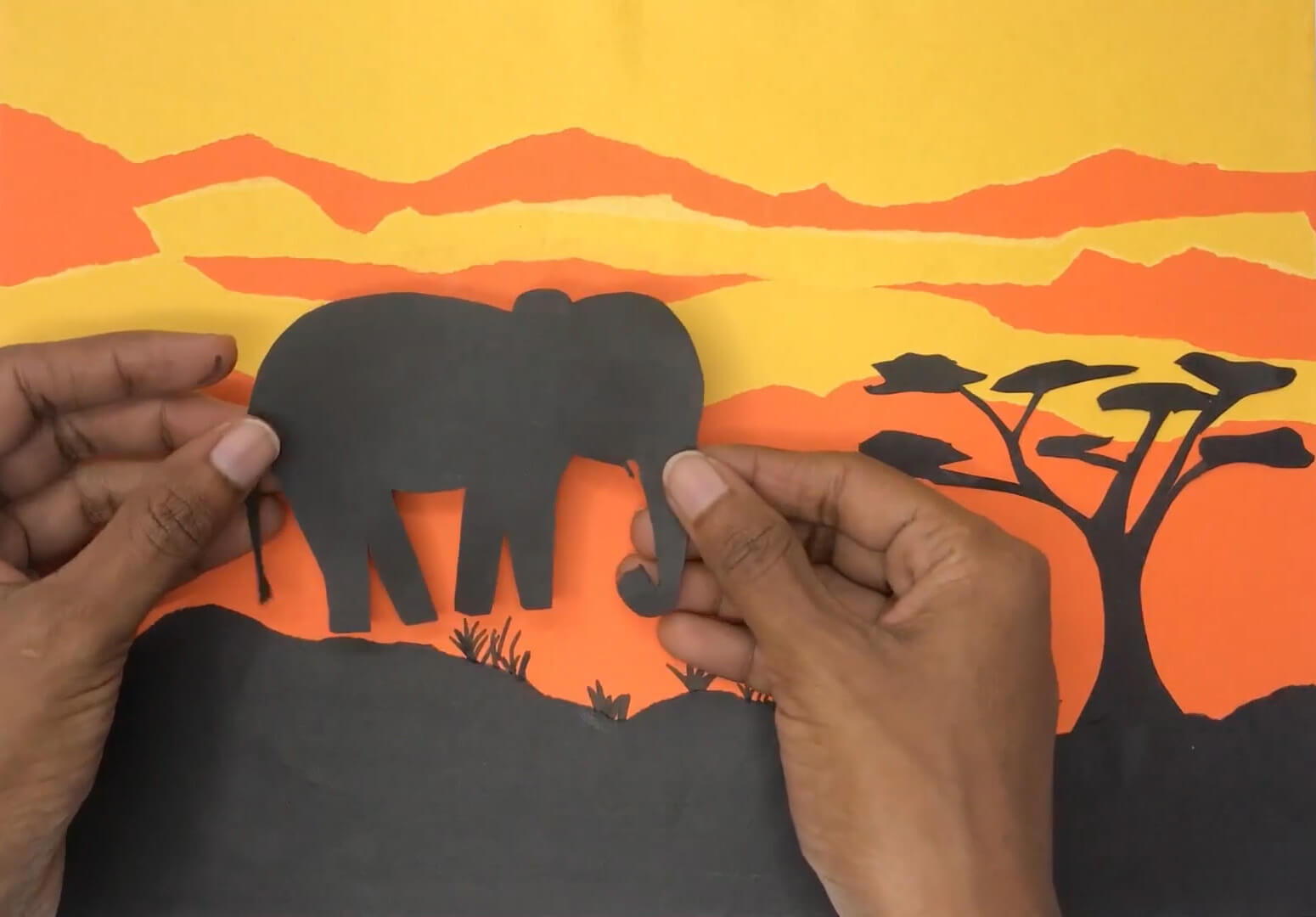The image showcases a meticulously crafted paper art collage set against a vibrant sunset background. The sky transitions from yellow to orange, with torn paper edges creating the effect of clouds and distant hills. In the foreground, a silhouette of a hilly terrain in black paper is adorned with delicate grass fronds and a uniquely curved tree, reminiscent of an African landscape. Dominating the scene is a black cutout elephant, held aloft by two brown hands with a rich, darker skin tone, thumb-side up, and positioned to place the elephant into the collage. The hands draw the viewer's attention and suggest the act of arranging or storytelling. The overall scene evokes the ambiance of a sunlit, serene afternoon, with the layered cardstock elements adding depth and texture to the tableau.